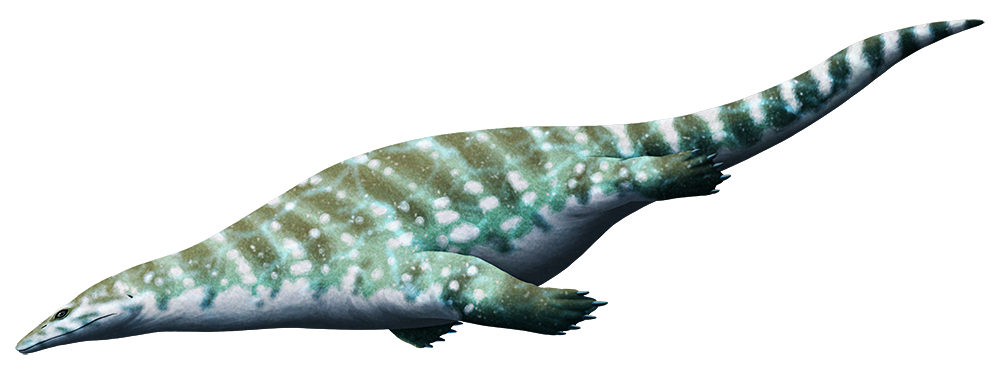The image depicts a prehistoric sea creature with its face oriented to the left and its tail extending to the right. The creature has a long, sharp face or elongated snout, reminiscent of both fish and porpoise anatomy, with a distinct, thin mouth line and a small, dark eye near the snout. Its body, which resembles that of a crocodile or alligator, is covered in a green, net-like pattern adorned with brown and white stripes that run across its length. The creature possesses four short limbs, each with six webbed toes. The tail is lengthy and tapers to a non-pointy end. The overall appearance suggests a fantasy or prehistoric nature, further accentuated by what appears to be an artistic rendering rather than a real-life photograph. This detailed depiction combines the attributes of aquatic and reptilian life forms, adding a mythical or space-like aesthetic to its patterning.